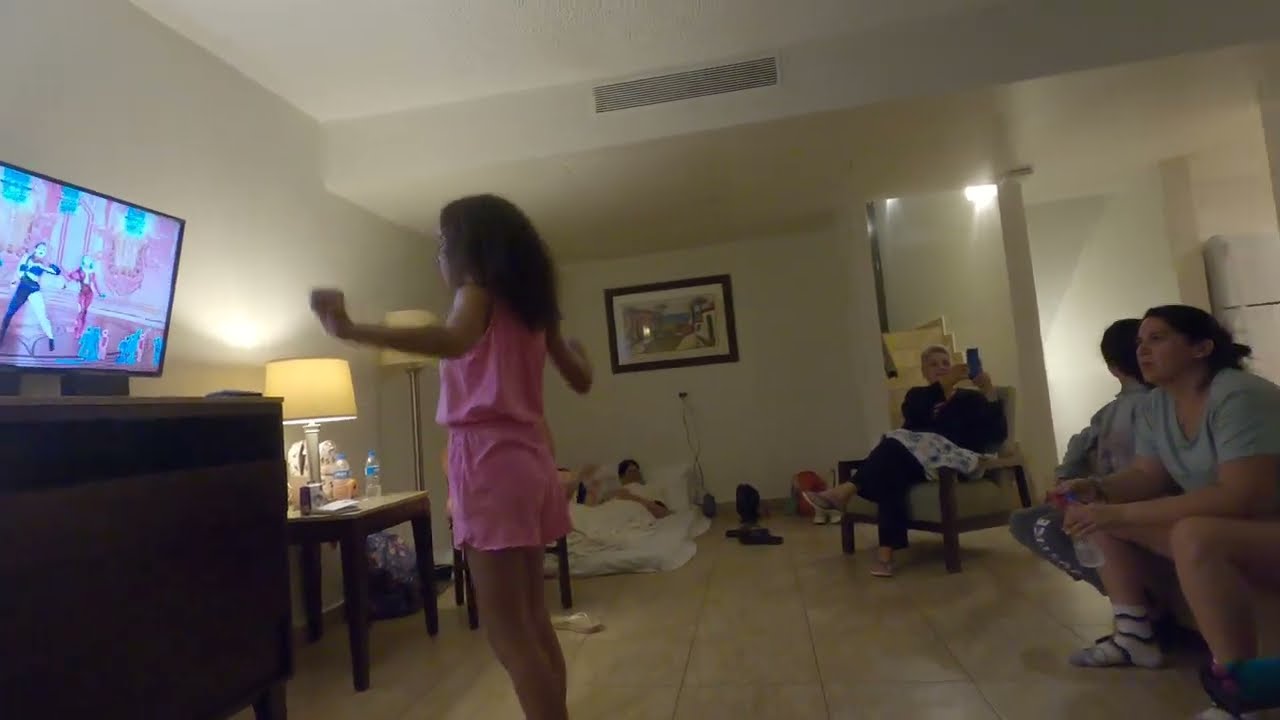The photograph captures a lively scene within a room of what appears to be an upscale, art deco-styled home with white walls and tasteful décor, including paintings and a well-lit lamp. The focal point is a young African-American girl dressed in a bright bubblegum pink tank top and matching shorts, energetically emulating dance moves from a cartoon displayed on the TV screen to her left. Her curly, shoulder-length hair bounces as she moves with her arms stretched out, immersed in the activity. 

To the right side of the frame, a somewhat blurred television reveals a cartoon with a pink background and animated characters, which seems to be the source of the girl’s dance inspiration. Nearby, an older woman with brunette hair in a bun sits in a brown and light brown chair, capturing the moment with a smartphone.

There are several other people in the room: one woman in a light blue t-shirt attentively watches the girl dance, while another person with their back turned sits beside her. In the background, a male figure relaxes on a makeshift bed on the floor, covered in white linens.

The setting provides a glimpse into a cozy family moment, highlighting the engaging activity of the young girl and the fond attention of her family members around her.